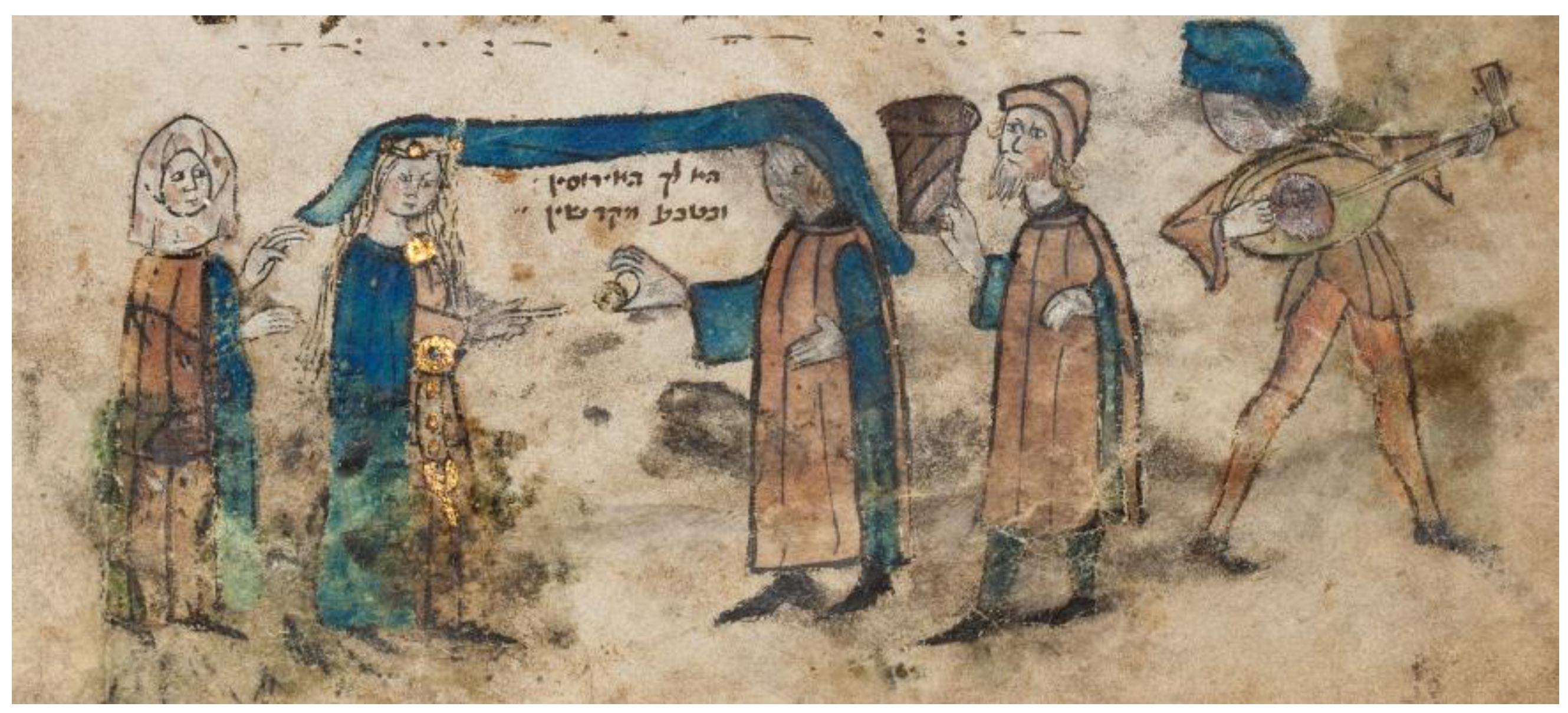In this aged and slightly damaged image, which exhibits characteristics of an old cartoonish watercolor drawing on light grayish parchment, there are five individuals prominently displayed, their interactions steeped in an aura of historical significance. The central figure on the left appears to be a queen, dressed in a regal light blue gown and a long brown cape, with an ornate headpiece marking her status. To her immediate right, a woman wearing a blue cloak and a cloth draped over her head, extending to a man beside her, seemingly part of a ceremonial exchange—he is dressed in an orange robe and his head is similarly covered, while he offers an item, possibly spices or a small bell. The scene also includes a man standing slightly to the right of center, holding a basket and adorned in an orange hat and cloak with pointy boots, hinting at his role as a servant or attendant. On the far right, a figure clothed in a blue turban and blurred attire, likely another servant, is playing a musical instrument, adding a layer of festivity or ritual to the scene. The image also contains a foreign script consisting of three to four words, enhancing the illustration's exotic and historical essence. The paper shows signs of wear, black smudges, and areas where the watercolor appears to have run or faded due to exposure to moisture over time.